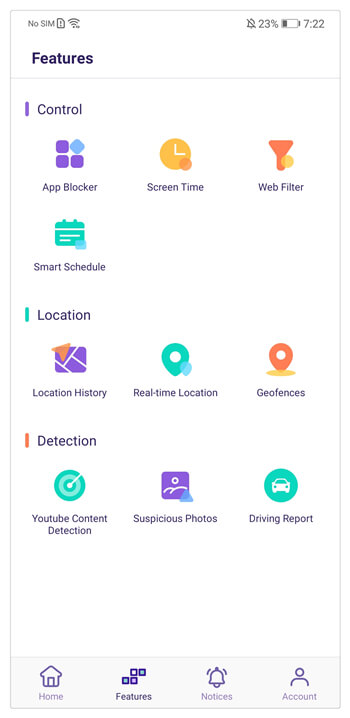This screenshot depicts a mobile device interface. Here are the detailed observations:

- **Top Left Corner**: Displays "No SIM" and the Wi-Fi signal icon.
- **Top Right Corner**: Shows the time as 7:22, with the battery level at 23%, and an alarm icon with a bell crossed out indicating alarms are disabled.
  
The entire background of the screenshot is white. Below the status indicators, the interface is divided into various sections:

1. **Features Section**:
   - The word "Features" is in bold above a gray line.
   
2. **Control Section**:
   - This heading is underlined with a purple line to its left and includes the following items:
     - **App Blocker**: Represented by four purple squares with a blue square tilted sideways.
     - **Screen Time**: Illustrated by an orange clock.
     - **Web Filter**: Depicted with an orange funnel.
     - **Smart Schedule**: Shown with a green briefcase icon.
   
3. **Location Section**:
   - Labeled with a green line to its left and contains the following sub items:
     - **Location History**: Indicated by a purple box with an orange arrow.
     - **Real Time Location**: Represented by a green location marker with a white circle in the center.
     - **Geofences**: Shown with an orange location marker and a white circle in the middle.
 
4. **Detection Section**:
   - Marked by an orange line on the left side of the section title "Detection" including:
     - **YouTube Content Detection**: Represented by a green radar icon.
     - **Suspicious Photos**: Illustrated by a purple box with white lines.
     - **Driving Report**: Depicted by a green circle with a white car inside.

This detailed breakdown offers a comprehensive view of each element displayed on the interface.